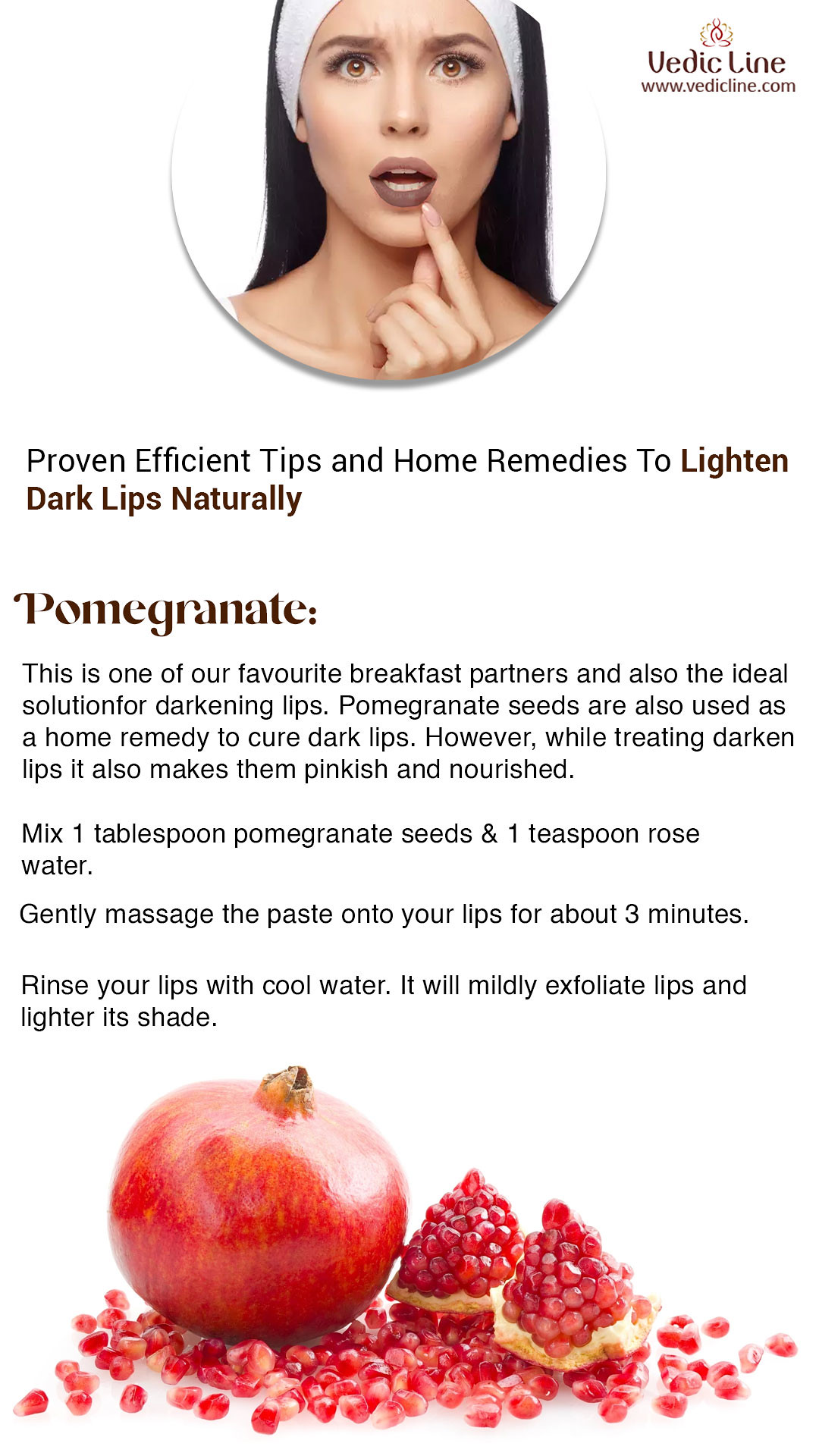This advertisement for VedicLine highlights a natural home remedy to lighten dark lips. At the top of the ad, a concerned woman wearing a nun’s headdress or possibly a towel, her hair long and black, applies a purple lipstick. To the right of her image is the VedicLine logo with the website, www.vedicline.com. Below her photo, the text reads: “Proven efficient tips and home remedies to lighten dark lips naturally. Pomegranate—one of our favorite breakfast partners and also the ideal solution for darkening lips. Pomegranate seeds are used as a home remedy to cure dark lips, making them pinkish and nourished. Mix one tablespoon pomegranate seeds with one teaspoon rose water. Gently massage the paste onto your lips for about three minutes, then rinse with cool water to mildly exfoliate and lighten your lip shade.” The advertisement’s bottom section features a vibrant pomegranate, both whole and split open, showcasing the seeds, which are integral to the suggested remedy. The overall color scheme includes browns, blacks, whites, and vivid reds and yellows from the pomegranate, enhancing the natural and wholesome vibe of the advertisement.